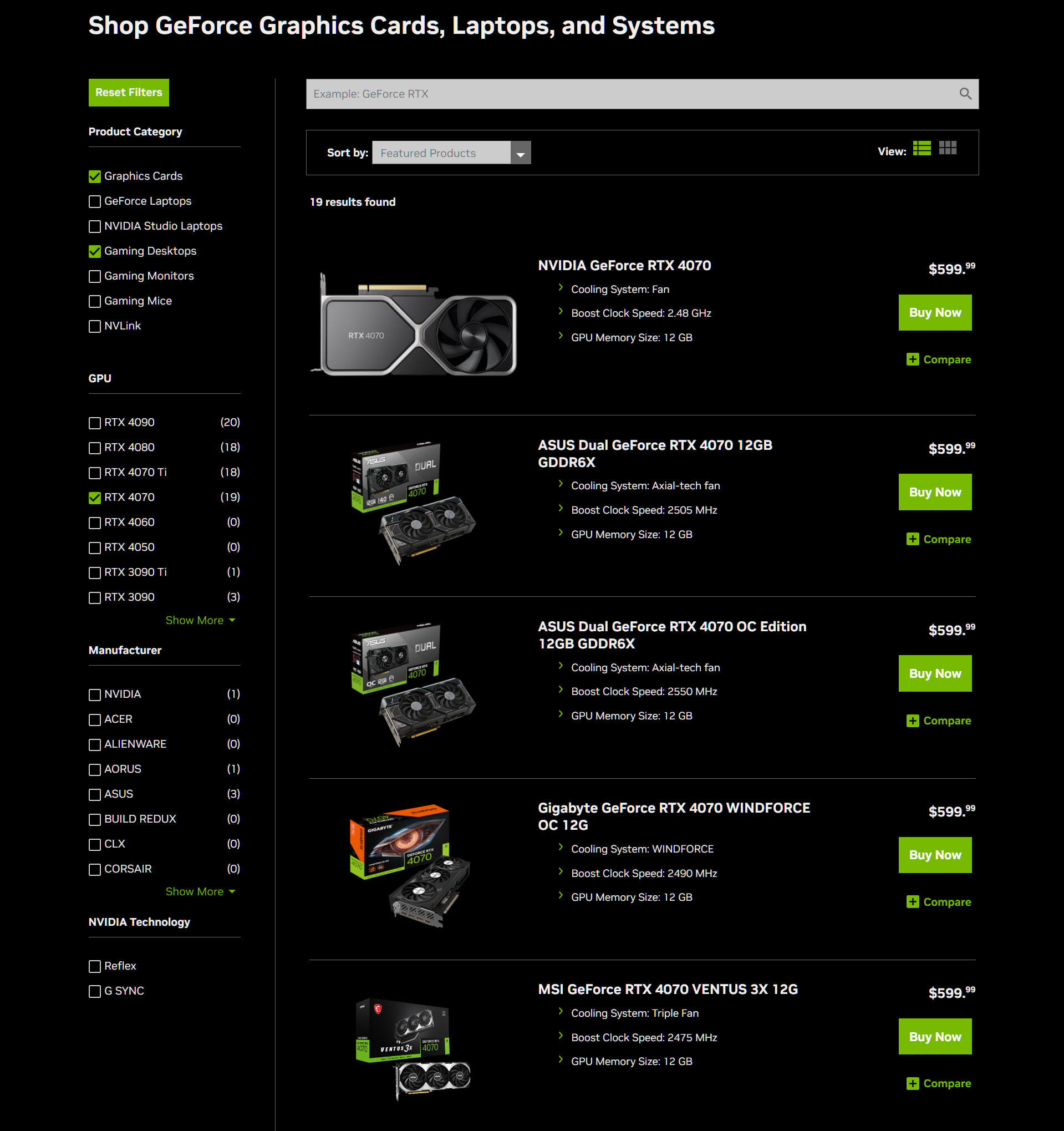The image is a screenshot of a product page from a website where various GeForce graphics cards, laptops, and systems are listed for sale. At the very top left of the screenshot, the section title reads "Shop GeForce Graphics Cards, Laptops, and Systems."

The featured products on the list appear to all be priced at $599. The first item is labeled "NVIDIA GeForce RTX 4070." The next product is an "ASUS Dual GeForce RTX 4070 12GB." Following this is another similar listing, also priced identically, labeled as "Gigabyte GeForce." Lastly, the list includes an "MSI GeForce RTX."

Each product seems to be a different brand or version of the GeForce RTX 4070 graphics card, all uniformly priced, giving potential buyers a variety of choices within the same price range. The image provides a clear view of the product offerings and their prices, giving users detailed information to compare while making a purchasing decision.